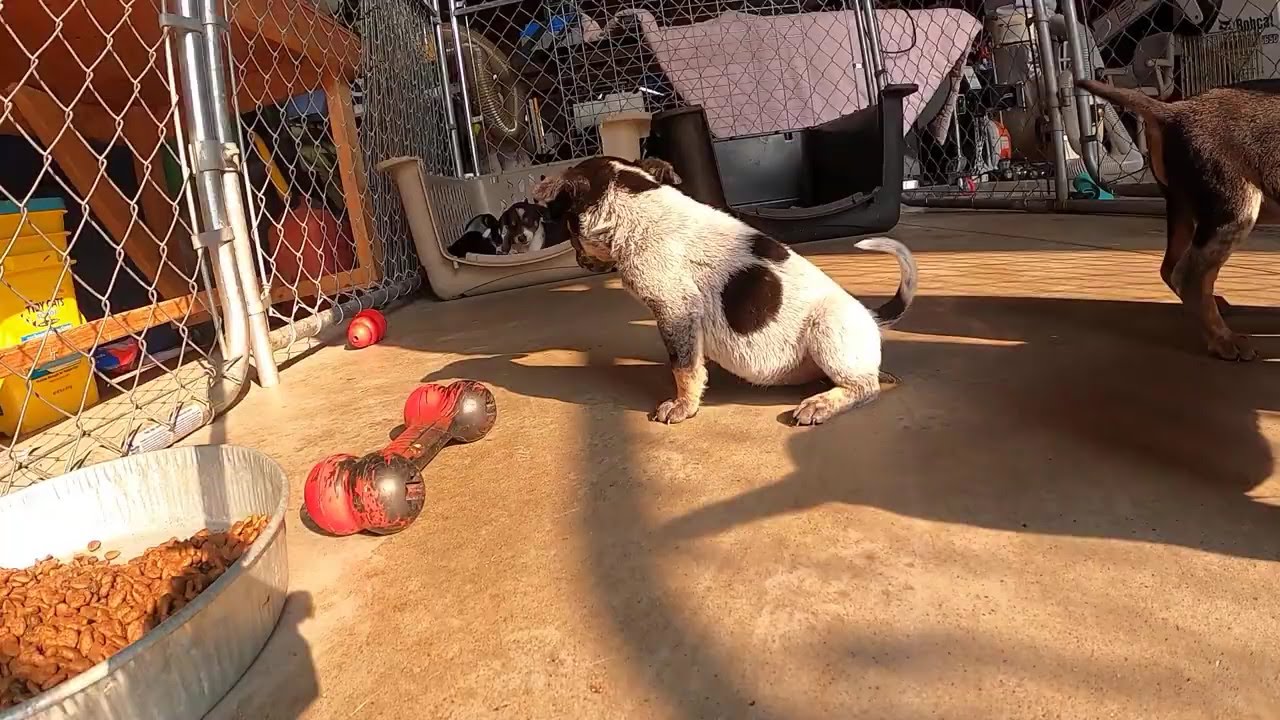This detailed image depicts a group of dogs, including adults and puppies, inside a metal chain-link pen situated on a concrete floor. In the background outside the pen, a large light pink blanket covers some objects, adding to the cluttered scene. To the left of the pen, a brown light wooden table holds a yellow container of what appears to be cat litter underneath it. 

Within the pen, the upper left-hand corner houses an upside-down dog carrier top containing puppies, including one with a brown face and a white spot on its forehead. Nearby, an empty black container is positioned next to a fat puppy with a white body, two large brown spots, and a brown head, lying next to a red and black toy bone. There's also a pan of food in a silver container in that same corner.

Another adult dog, predominantly white with brown spots, can be seen along with other brown short-haired dogs, all in various states of rest and play. The presence of food, water, and toys, including another red toy, suggest efforts to keep the dogs occupied and contained, possibly to avoid damage and mess in an indoor environment. The overall scene gives the impression of a makeshift kennel area designed to manage a boisterous group of unhousebroken puppies and their caretakers.